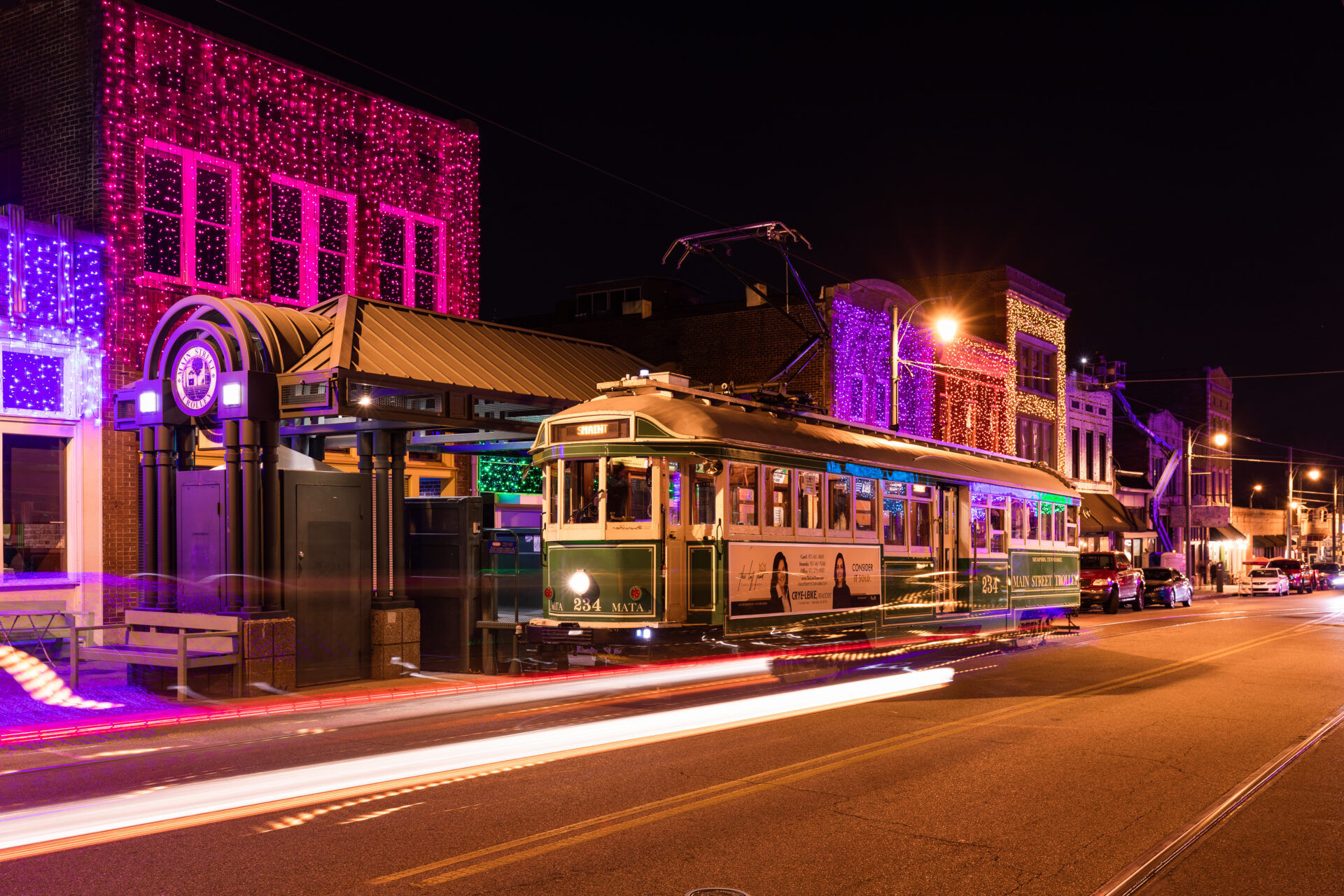The nighttime street scene is captured in a landscape orientation, with a diagonal perspective emphasizing the angled composition. The sky is pitch black, dominating the top of the photo. A green and cream-colored trolley, adorned with windows on its upper half, traverses the street, its vintage design underscored by the visible overhead wires powering it. The trolley emits a beam of white light, which slices through the dark atmosphere, highlighting its path. Behind the trolley, on the left side, stands a loading station with a distinct black and metal arch. 

Illuminating the scene are vibrant neon lights from the street's storefronts, creating an eclectic glow. One building features a light purple facade, while another is lit with pink lights, suggesting a festive array of Christmas decorations. The surrounding architecture consists of old square buildings, three to four stories tall, giving a historic feel to the scene. 

On the right, a series of parked cars line the street, adding to the urban tableau. Although the streets are devoid of people, the vivid LED lights and colorful facades suggest shops, restaurants, and bars are nearby. The combination of these elements, alongside the trolley numbered 234, paints a lively, albeit quiet, nocturnal cityscape.